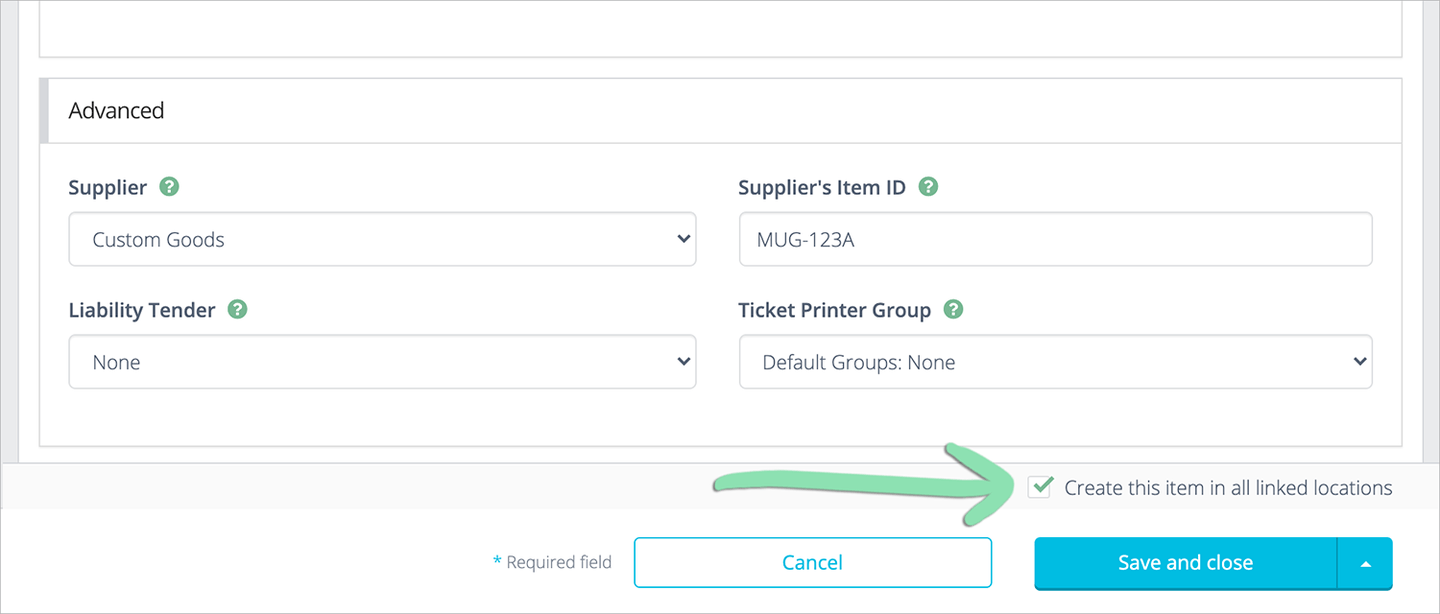The screenshot showcases an advanced selection area on a website with a white background. The main section is structured into a two-by-two grid containing four selection criteria. Each criterion is labeled and accompanied by a green circle with a white question mark icon for additional information.

1. **Top Left - Suppliers:** The dropdown menu is labeled "Suppliers" and is currently set to "Custom Goods."
2. **Top Right - Supplier's Item ID:** This criterion is a text input field labeled "Supplier's Item ID," with the value entered as "MUG-123A."
3. **Bottom Left - Liability Tender:** The dropdown menu labeled "Liability Tender" is set to "None."
4. **Bottom Right - Ticket Printer Group:** The dropdown menu labeled "Ticket Printer Group" is set to "Default Groups None."

Below the selection grid, there is a checkbox labeled "Create this item in all linked locations," which is checked and indicated by a green checkmark. 

Further down, to the left of the checkbox and the buttons, a blue asterisk indicates a required field. The bottom right corner features two buttons: a "Cancel" button with a white background, light blue outline, and blue text, and a "Save and Close" button with a light blue background and white text.